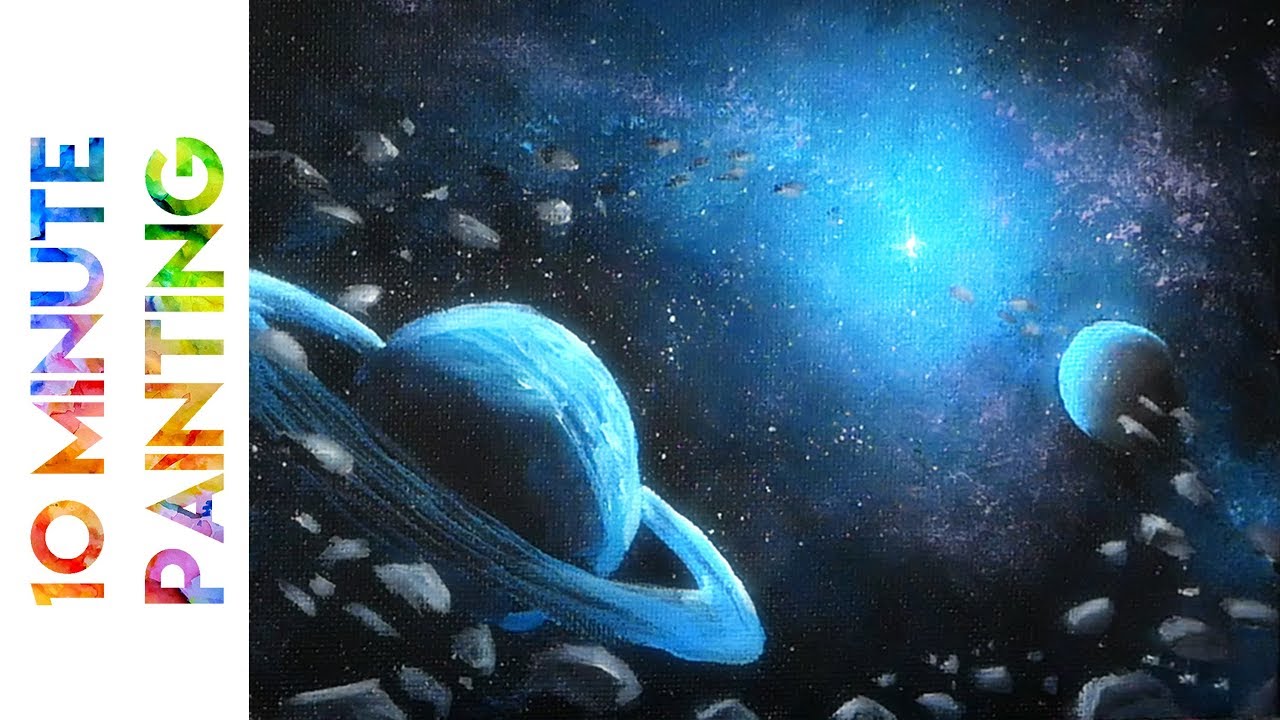On the left side of this image, in a vibrant, rainbow watercolor style, vertical block lettering reads "10-Minute Painting." The words ascend from bottom to top, with each letter in a different color. To the right, the artwork illustrates an expansive view of space, dominated by shades of blue and black. In the bottom left corner, there's a ringed planet that might be Saturn, characterized by its blue hue, possibly reflecting the light of a distant star. Numerous asteroids and rocks float through the scene, suggesting a dynamic and textured cosmos. On the right, another smaller planet appears, possibly Earth. Scattered throughout the painting are myriad white specks representing distant stars. The upper right corner features a particularly bright star, casting a radiant glow over the composition. Overall, the painting vividly captures the ethereal beauty of the Milky Way galaxy with its dark corners and luminous highlights.